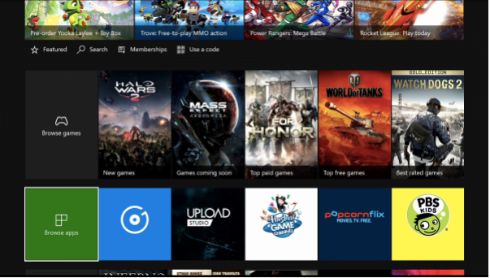The displayed image captures an Xbox app interface showcasing a variety of games and apps organized in a bookshelf-like arrangement. Dominating the central section is the "Browse Games" category, featuring visible titles such as Halo Wars 2, Mass Effect, For Honor, World of Tanks, and Watch Dogs 2. Adjacent to this is the "Browse Apps" section, hosting a collection of applications. One app with a blue background and a central circular icon stands out, followed by Upload Studio, an unidentified game with a smaller icon, Popcorn Flicks, and PBS Kids. The PBS Kids app is particularly eye-catching with its bright yellow background, featuring a smiling child with green skin and the PBS Kids logo prominently displayed. At the top of the interface, there are four additional game icons, though their titles are not discernible. Below these are options for "Featured," "Search," "Memberships," and "Use a Code," offering various functionalities within the app. The harmonious arrangement and vibrant colors, especially the PBS Kids app, make it markedly noticeable.